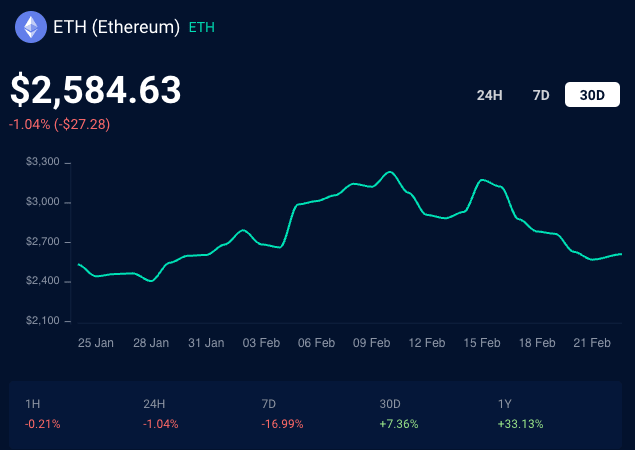In this image, there is a detailed screenshot of a cryptocurrency price graph specifically for Ethereum (ETH), displayed in the upper left-hand corner. The title "ETH" is followed by the notation "Ethereum" in parentheses. Beneath this title, the current price of Ethereum is listed as $2,584.63. Adjacent to this figure, on the right, are options to adjust the graph’s timeframe to either 24 hours, 7 days, or 30 days. On the left side, there is an indication of a recent price change: a decrease of 1.04%, equivalent to a loss of $27.28.

The accompanying graph spans a date range from January 25th to February 21st. The vertical axis on the left side shows a scale ranging from $2,100 at the bottom to $3,300 at the top, indicating the price fluctuations within this period. Below the graph, a summary of percentage changes is displayed for various durations: 1 hour, 24 hours, 7 days, 30 days, and 1 year. The percentages for the shorter time periods (1 hour, 24 hours, and 7 days) are shown in red, denoting negative changes. In contrast, the percentages for the longer time periods (30 days and 1 year) are in green, reflecting positive growth.